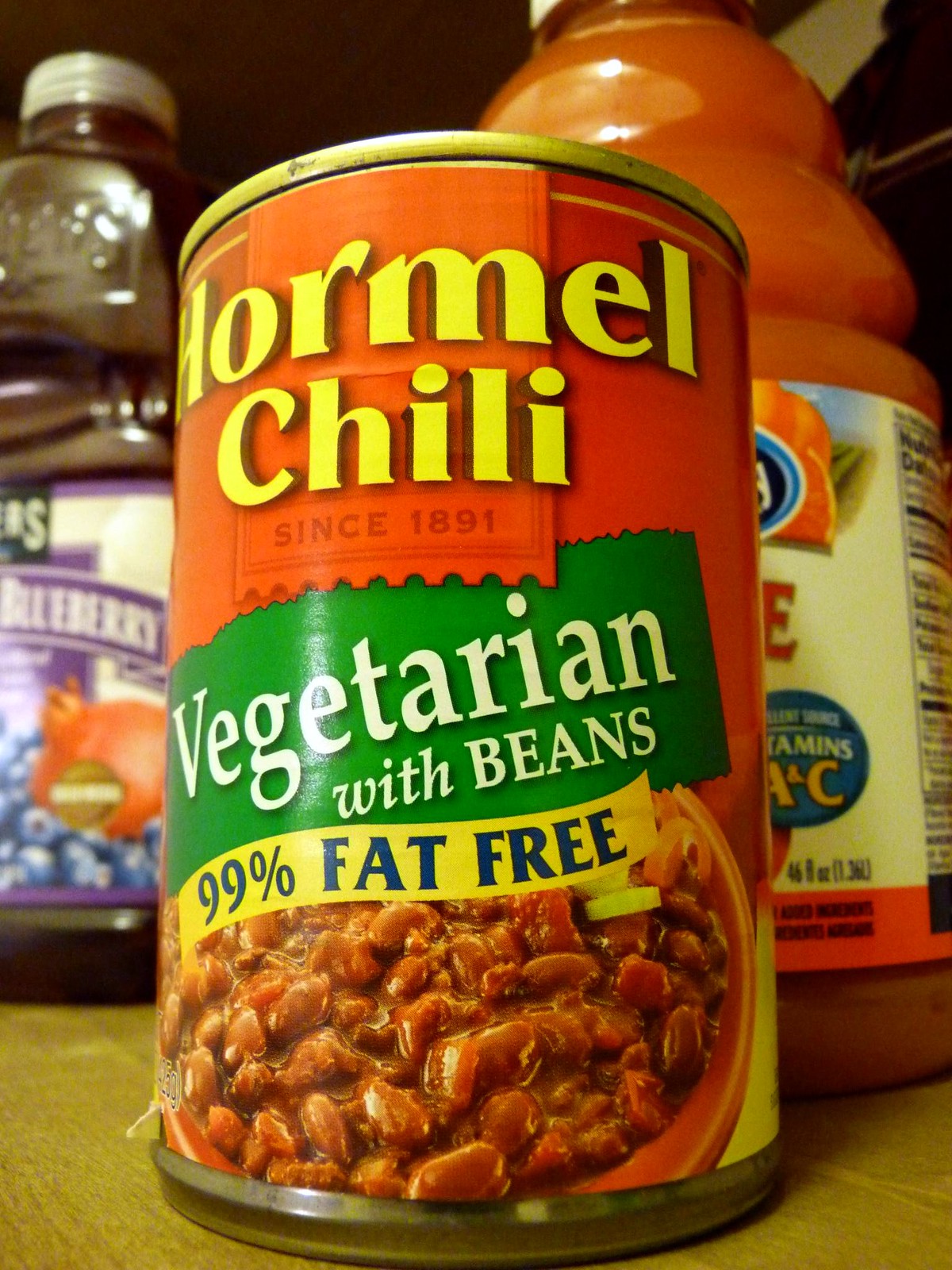The photograph features a collection of beverages and a canned food product against a neutral background. On the left side of the image, there stands a clear glass bottle filled with a deep purple liquid, likely blueberry juice, judging by the detailed label. The label is adorned with vibrant images of blueberries and pomegranates and prominently displays the word "Blueberry." To the right of this bottle, there is a plastic bottle containing a pink-hued juice. The visible portion of its label highlights the nutritional content, specifically noting the presence of vitamins A and C.

At the center, and clearly the focal point of the image, is a can of Hormel chili. The can is marked with the brand's name "Hormel chili" in bold yellow letters. Below the brand name, the text "Since 1891" is displayed, establishing the product's long-standing history. A green banner on the can indicates the chili is "Vegetarian with Beans," and beneath this, a yellow banner asserts the product is "99% Fat-Free." The label features a serving suggestion, illustrating a hearty bowl brimming with chili, adding a visual appeal to the product's presentation.